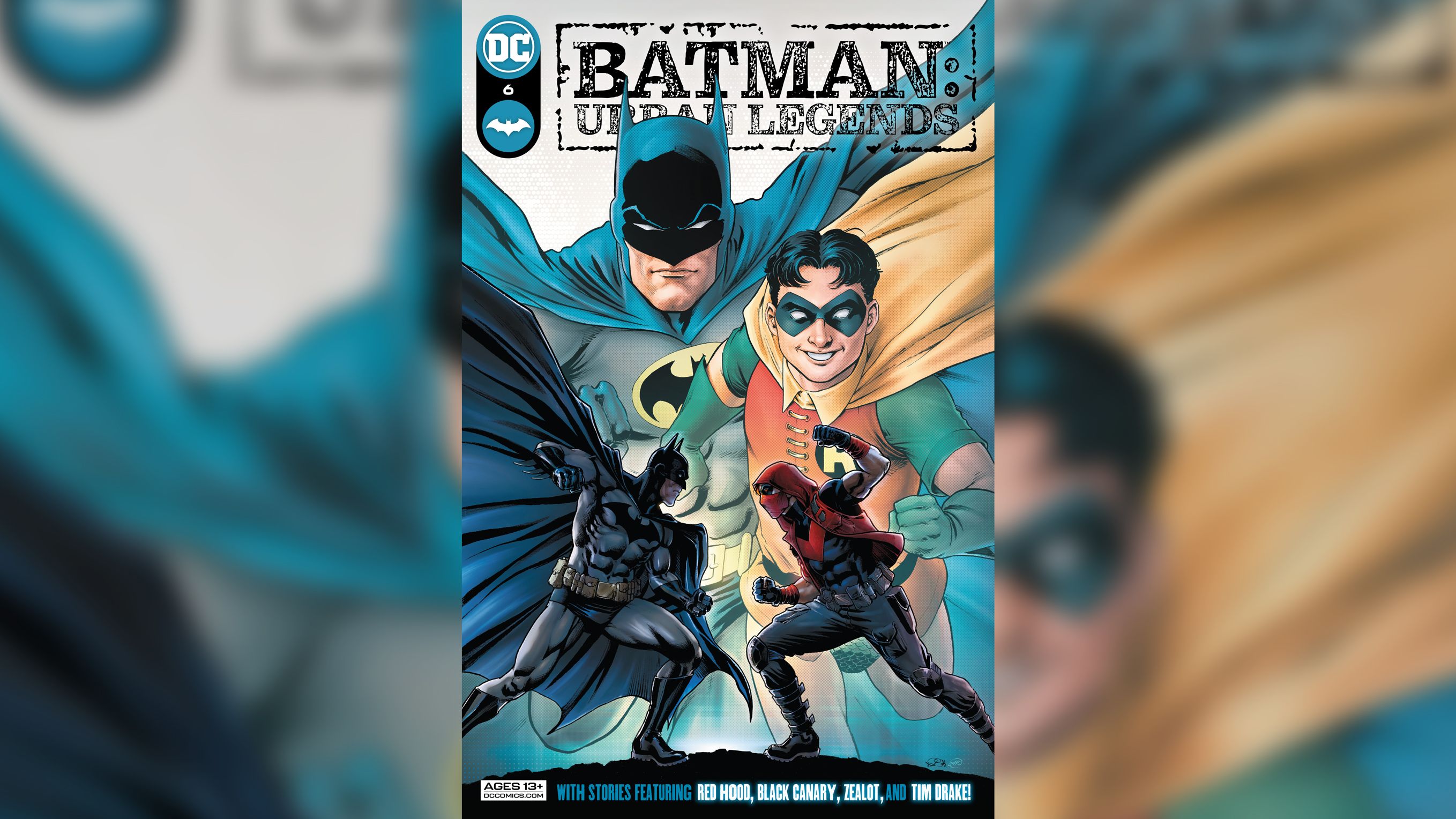The comic book cover of "Batman: Urban Legends" by DC Comics prominently features Batman and Robin in dynamic poses. Batman, dressed in his classic blue cape, black mask, and gray suit adorned with the iconic Bat emblem surrounded by a yellow ellipse, is positioned powerfully with his arms spread wide. Robin stands to Batman's right, wearing a black mask, yellow cape, green sleeves, and a red vest emblazoned with an 'R'. Both characters dominate the background. In the foreground, a battle scene unfolds where a smaller, fully black-clad Batman confronts Red Hood (Jason Todd), who is distinguished by his full-face red mask and matching red body armor. The issue, marked as number 6 in the series, is highlighted in the upper left corner below the DC logo and a smaller Bat symbol. The cover also indicates that this comic is suitable for readers aged 13 and up and features additional stories involving Red Hood, Black Canary, Zealot, and Tim Drake.